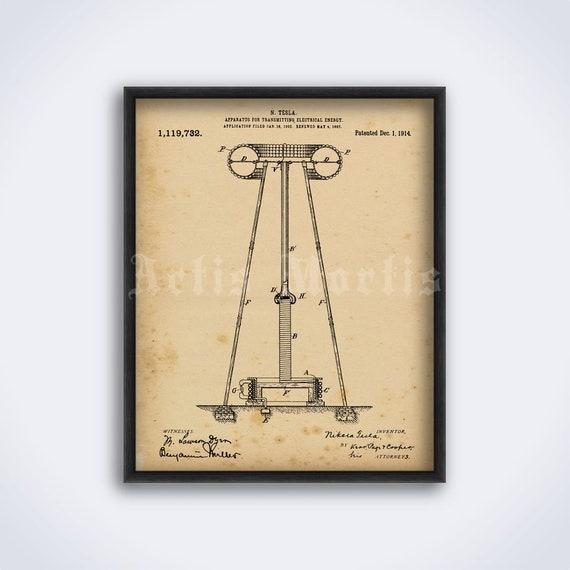In a light gray rectangular frame hanging on a presumably museum wall during daytime, there is a prominently displayed, aged and decaying beige document, evoking an antique look with noticeable dirt marks particularly along the left edge and bottom. This document, appearing as an old patent drawing by Nikola Tesla, is depicted with a black illustration at its center, suggesting a complex apparatus, possibly a pendulum or electrical transmitter. The intricate details include potential wheels and weighted components, although the precision of the invention remains uncertain due to the faintness and small size of the descriptive text. Above the illustration, "N.Tesla" is inscribed, emphasizing the inventor's contribution. Below the drawing, various signatures are present, likely of the patent officials, while the top left corner bears the patent number "1,119,732" and the top right denotes the issue date as "December 1st, 1914."